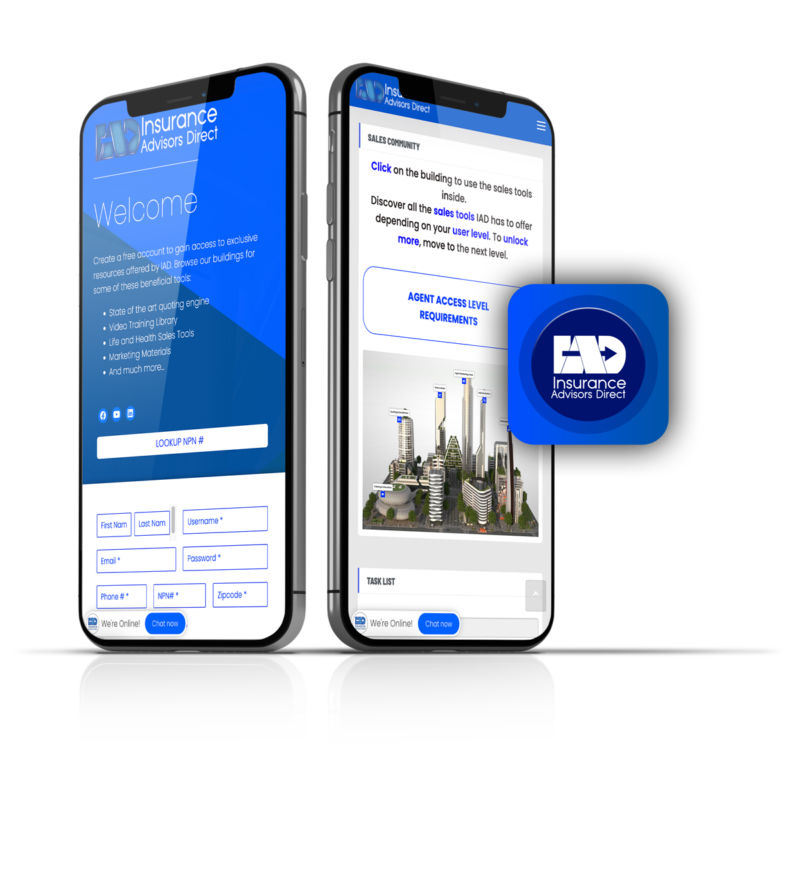In this image, there are two upright cell phones positioned side by side, with one facing the left and the other facing the right. The left cell phone displays an open insurance application. The app welcomes users and encourages them to create a free account to access exclusive resources offered by "Insurance Advisory Direct" (IAD). These resources include a state-of-the-art quoting engine, a video training library, life and health sales tools, marketing materials, among other benefits. The app interface also has fields for entering personal information such as first name, last name, username, email, password, phone number, and zip code.

The right cell phone shows a different screen, presumably related to access level requirements or a task list tied to the same insurance company. Both phones feature a small blue "Chat Now" button in the bottom left-hand corner for live assistance. The bottom right corner of each phone displays the IAD logo, which consists of the letters "I," "A," and "D" in white, capital letters with an arrow pointing to the right. This branding signifies "Insurance Advisory Direct."